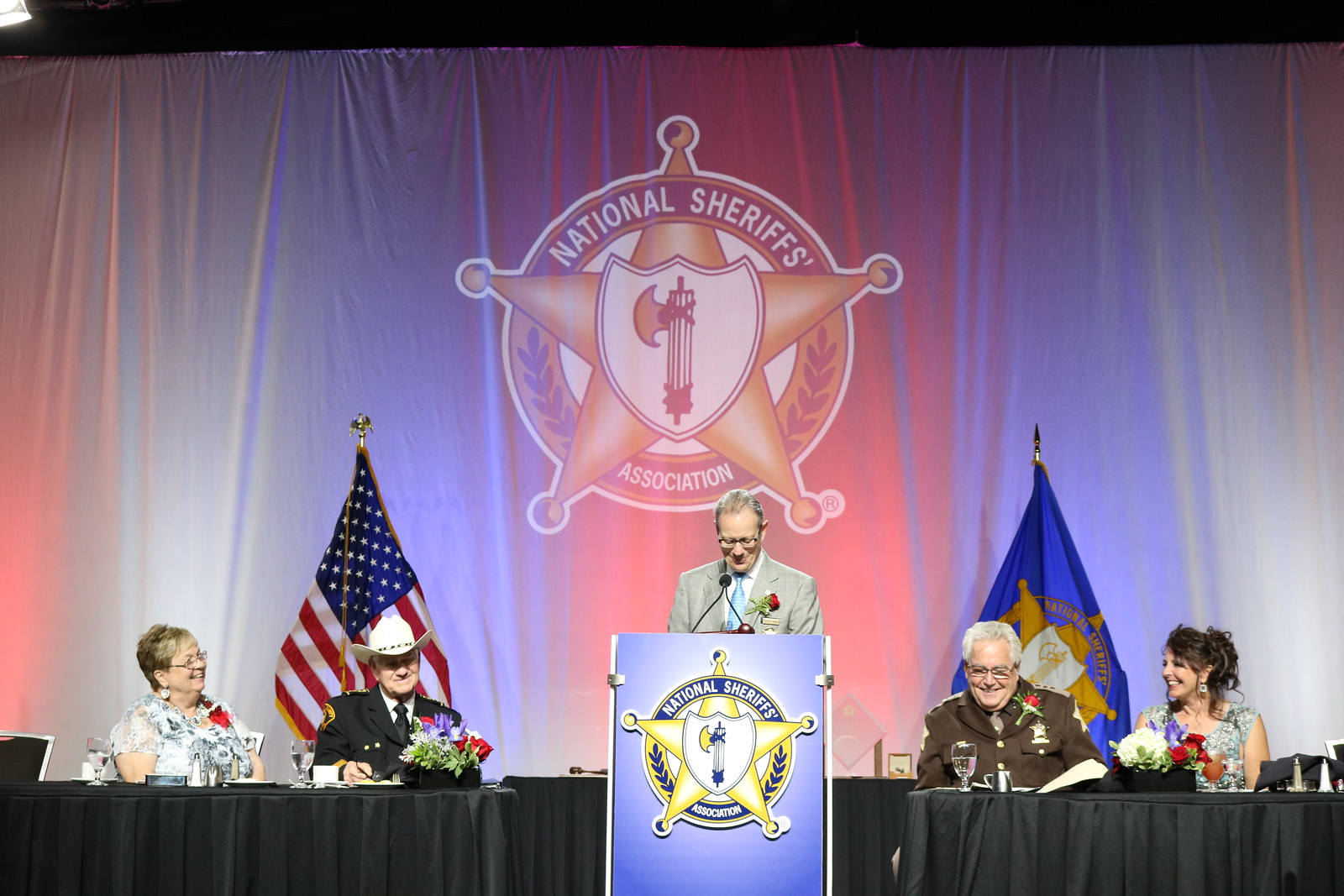The image captures a vibrant banquet scene set against a backdrop curtain featuring a projected emblem of the National Sheriff's Association, a circle with a gold star at its center, reminiscent of a traditional sheriff's badge. Below this projection stands a blue podium adorned with the same emblem. A man in a beige suit with a light blue tie and a rose corsage is speaking at the podium, which is equipped with a microphone. He is flanked by two American flags on the right and two blue flags with the National Sheriff's Association emblem on the left. Seated to his left are a man and a woman, and to his right, another man and woman, all of whom also wear rose corsages. The tables in front of them are decorated with flowers and drinks. Notably, one man with a cowboy hat adds a touch of regional flair. The scene exudes a lighthearted atmosphere, as it appears the speaker just made a joke, eliciting smiles and laughter from the attendees.